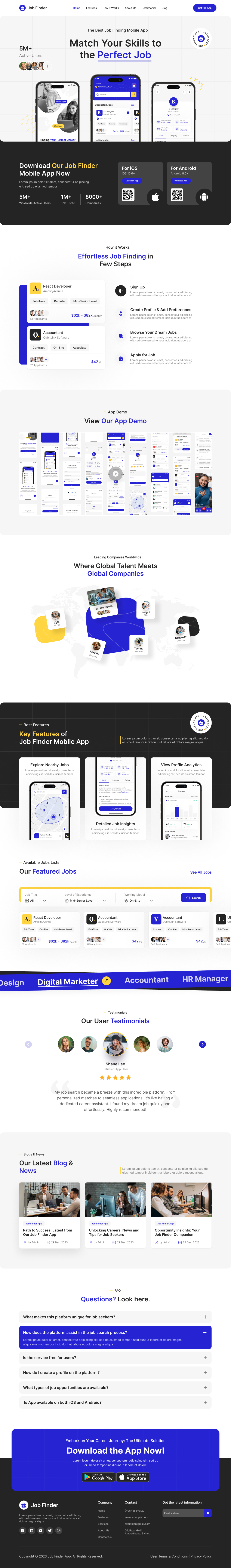This is a screenshot of a highly distorted app interface, predominantly featuring hues of light gray and white. In the top left corner, a cobalt blue circle is followed by black text. The upper middle section contains additional smaller black text, succeeded by a blue ovular button located at the top-right corner. Below this, there's an illegible section of text.

Central to the image, bold black text states "Match your skills to the," followed by blue text saying "perfect job." Just below this text, the top third of three different cell phones is visible, aligned side by side, each displaying various screens.

Underneath the cell phones, a black rectangular banner stretches horizontally from left to right. On the left side of the banner, white text reads "Download" followed by yellow text that states "our job finder." This is immediately followed by more white text: "mobile app now." To the right of this banner are two additional rectangles containing text that is too small and distorted to decipher.

Further down, two primarily white rectangles with black and some blue text are visible. They convey messages about "effortless job finding in a few steps," as well as "view our app demo and different screenshots of the app demo." The very bottom of the screenshot contains additional app download information, urging users to "download the app now."